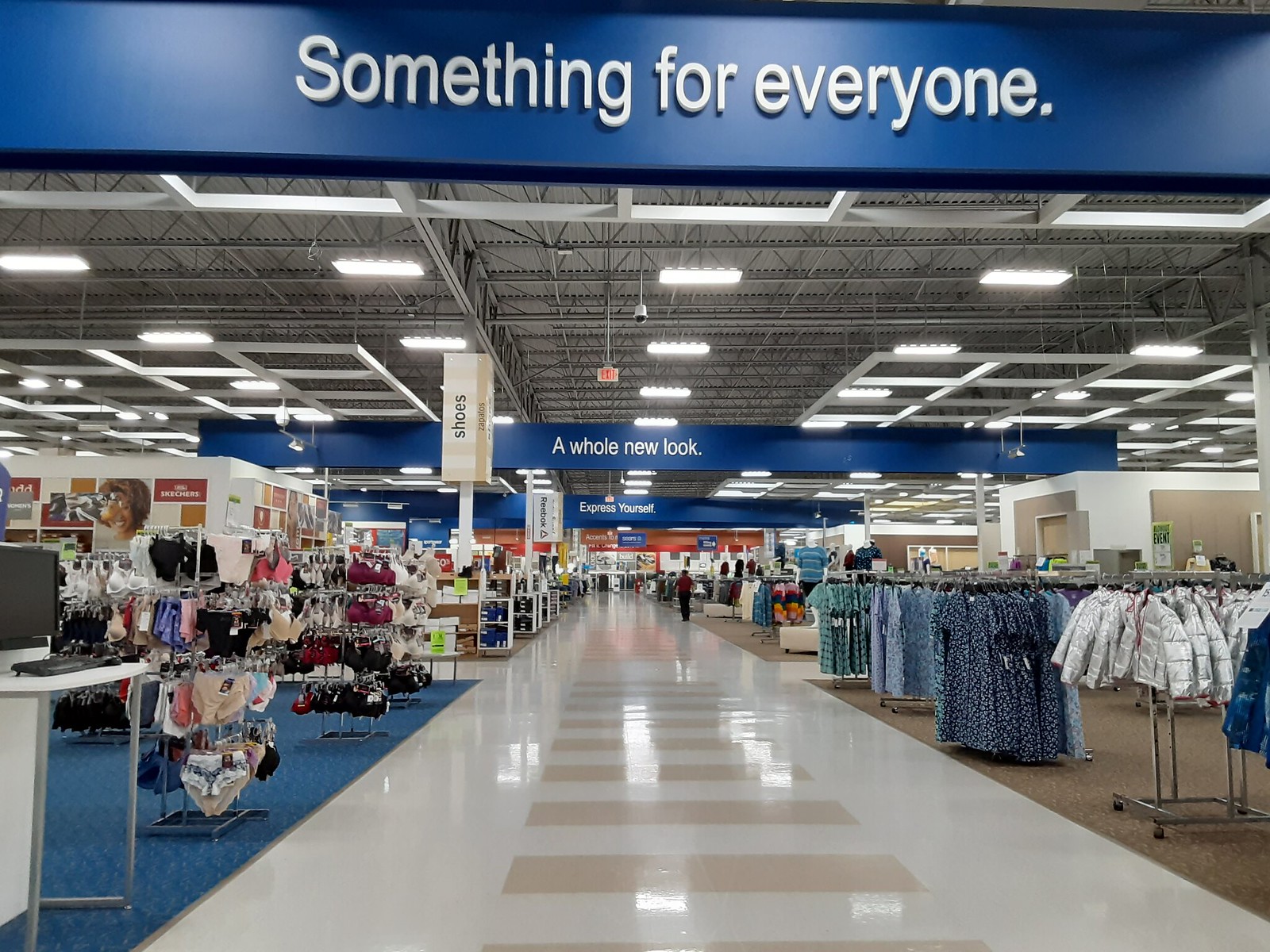This color photograph showcases the interior of a large retail store. At the top of the image, there's a prominent blue sign with white text that reads "Something for Everyone." In the distance, another similar sign can be seen, bearing the message "A Whole New Look," while a third sign is visible further back but too small to be legible. The ceiling of the store is grey and exposed, revealing an array of wires and numerous fluorescent lights.

Below the ceiling is a white walkway, accented with green horizontal lines or steps. This walkway is flanked by multiple displays of clothing items. On the right side of the image, there are blue dresses, green tops, and short white jackets. On the left side, smaller shelving areas are filled with what appears to be underwear. A light grey desk or shelving area is situated at the far left corner of the photograph. In the center, distant and tiny images of shoppers can be seen, giving a sense of scale and activity within the store.